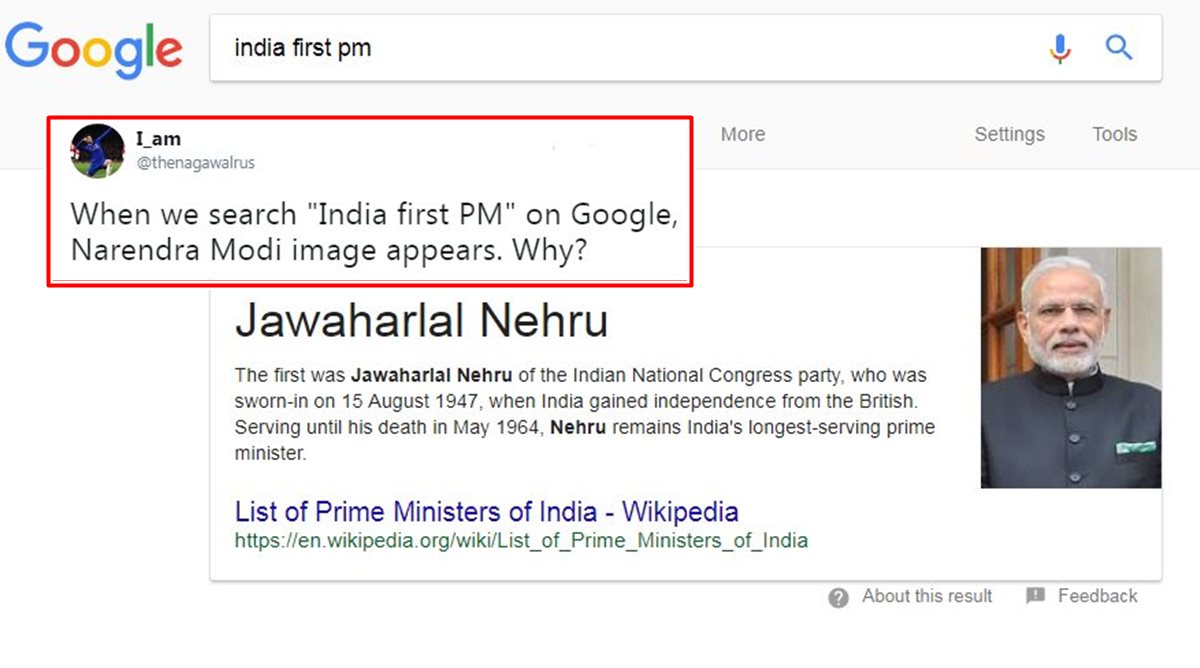This image is a screenshot of a Google search result for "India first PM," with a user's comment overlaying the screen just below the Google search bar. The comment is enclosed in a red text box and features the handle @TheNagaWalrus. The comment reads: "When we search 'India first PM' on Google, a Narendra Modi image appears. Why?" The screenshot incorrectly shows an image of Narendra Modi instead of Jawaharlal Nehru, who was the first Prime Minister of India. Nehru, a member of the Indian National Congress Party, was sworn in on August 15, 1947, following India's independence from British rule, and served until his death in May 1964, making him India's longest-serving Prime Minister. Accompanying this error, there's a picture of a man with white-gray hair and a short white-gray beard with a mustache, wearing a black button-up jacket. The image also contains a Wiki link labeled "List of Prime Ministers of India, Wikipedia."